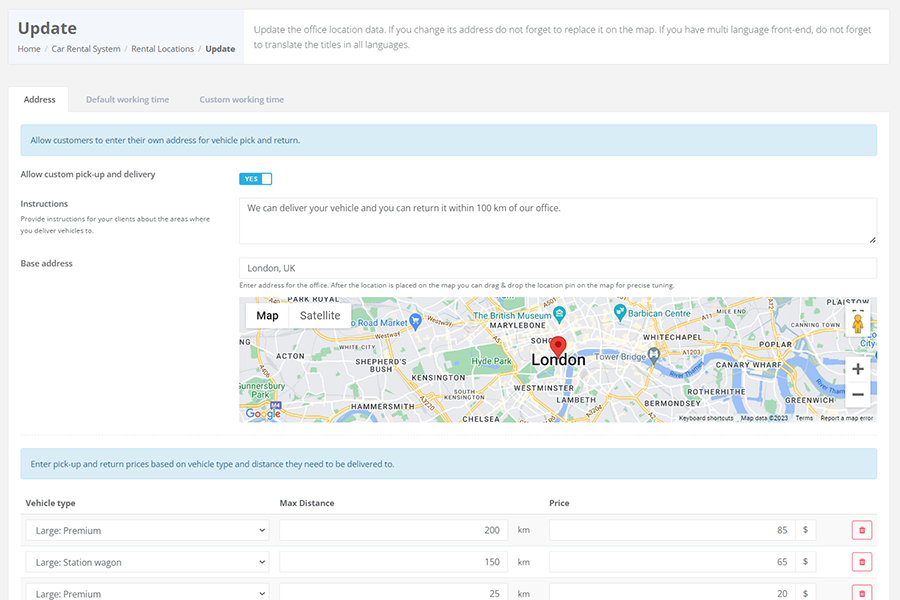The image displays a user interface of a car rental website, specifically focused on rental locations. The webpage highlights an update concerning available rental locations in central London. Visible at the bottom of the interface is a section where users can select the type of vehicle they wish to rent. The website clearly aims to facilitate the process of renting cars in London with a streamlined and user-friendly layout.